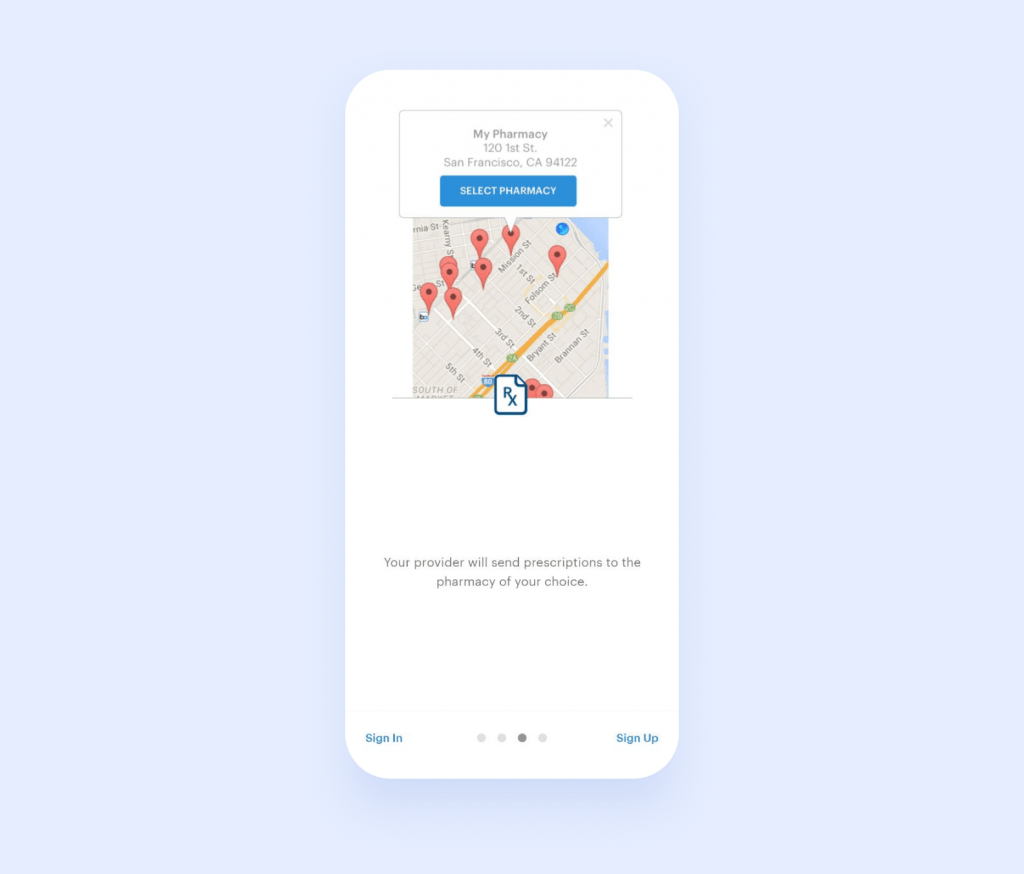This is a detailed caption for the image described:

The image is a diagram showcasing the screen of a mobile device. At the center of the screen is a Google Map image depicting a city that appears to be San Francisco. The map features multiple red location pins, each representing different "My Pharmacy" locations. One of the pins, located near Mission Street, is highlighted with a text box extending from it. The text box states: "My Pharmacy, 100 1st Street, San Francisco, CA 94122." Directly below this information, there is a prominent blue button with the words "Select Pharmacy" written in white.

At the bottom of the screen, there are two lines of text providing additional instructions: "Your provider will send prescriptions to the pharmacy of your choice." At the very bottom of the window, there are two options: "Sign In" on the left and "Sign Up" on the right. Between these options, there are four grey dots aligned horizontally.